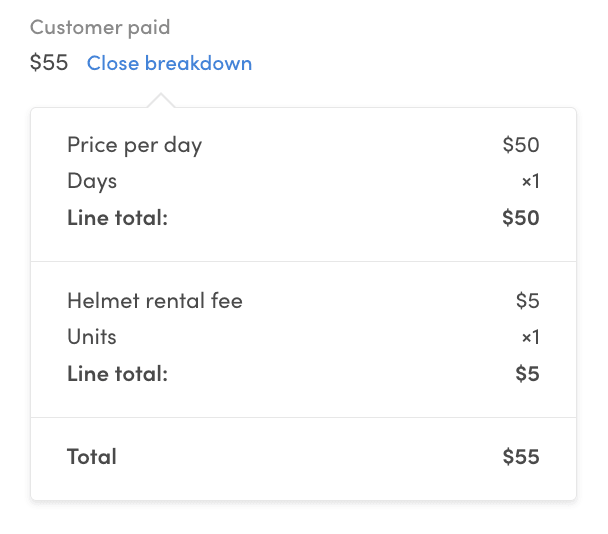A clean, simple visual featuring a white background with grey and blue text. On the left-hand side, the heading reads "Customer Page" accompanied by a dollar sign and the figure "55". To the right, in bright blue, the title "Closed Breakdown" is displayed. The breakdown is as follows:

- **Price per day:** $50
- **Days:** x 1
- **Line Total:** $50
- **Helmet Rental Fee:** $5
- **Number of Units:** x 1
- **Line Total:** $5

Below this, the **Total** is displayed as $55.

The overall layout is divided into three sections, separated by very faint blue lines. Each section is delineated with a line across after each total and at the top and bottom of the breakdown. A subtle detail is observed: as you trace the top line from the left, it dips slightly around the "R" in "Breakdown" before resuming its horizontal path.